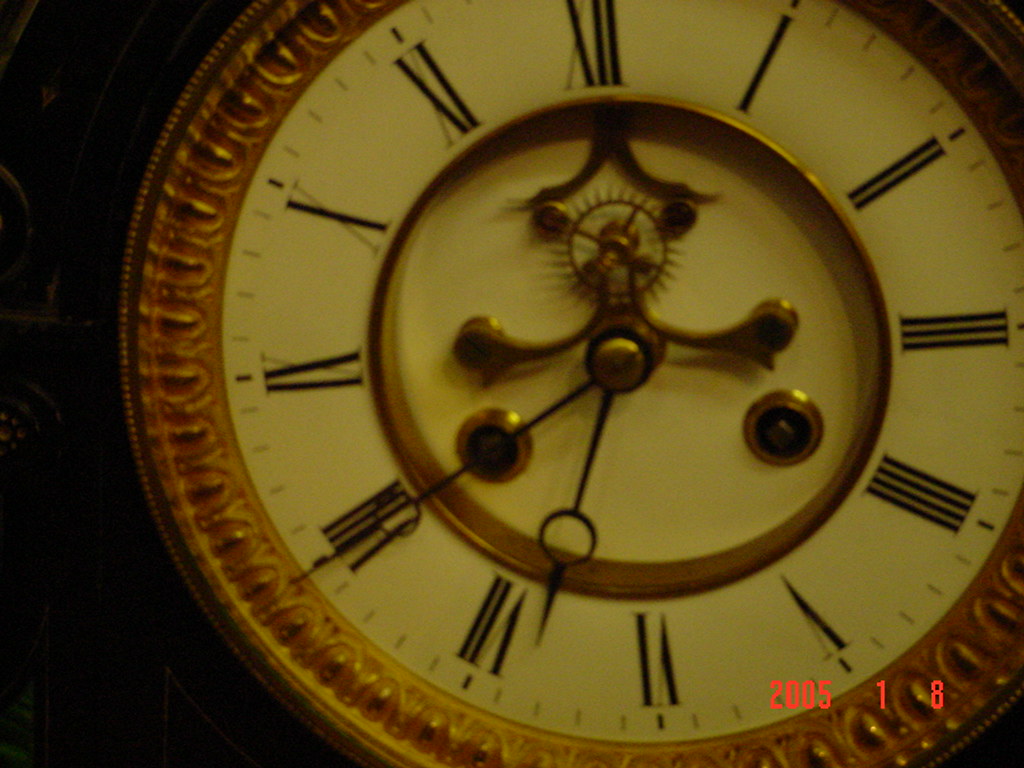This detailed, close-up image captures an antique wind-up clock with a date stamp reading "2005-18" in red, located at the lower right corner of the slightly rectangular frame. The clock face, white from age but now yellowed, is adorned with black Roman numerals and is encircled by ornate, gold inscribed rectangles with arches, enhancing its antique aesthetic. At the center, an exposed gear occupies the 12 o'clock position, showcasing intricate brass mechanisms. Two brass circles, designed for key insertion to wind the clock, are prominent features. The black hands of the clock are intricately designed, with the hour hand distinguished by a large, open circle near its pointed tip. The backdrop is a stark black, emphasizing the clock's vintage elegance. The time displayed is 20 minutes to 7.